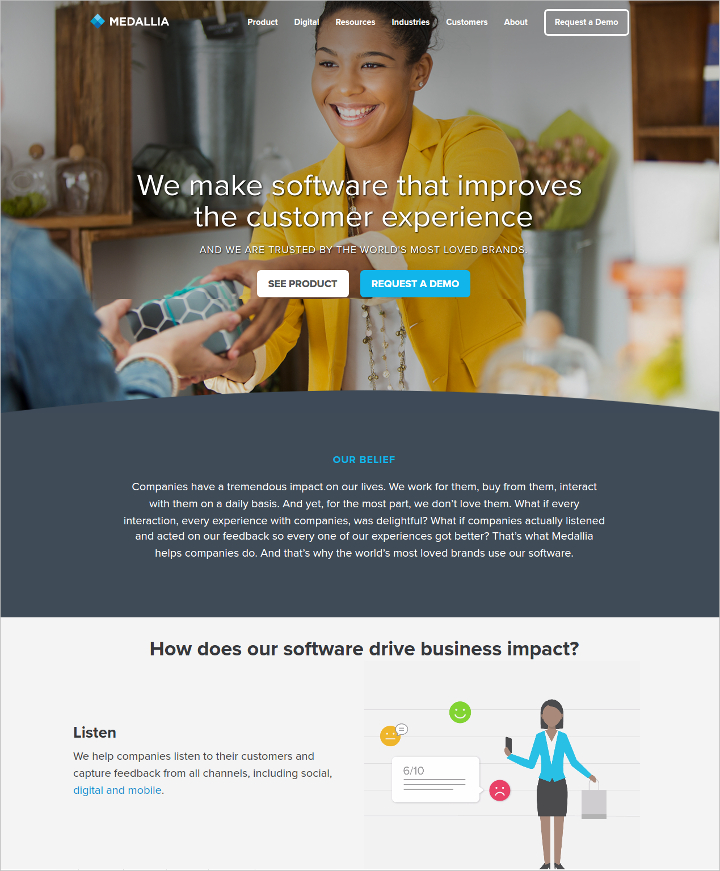The image depicts the homepage of Medallia's website. Medallia is spelled M-E-D-A-L-L-I-A, and their brand logo comprises a square containing four smaller squares, each shaded in different hues of blue. The logo, when tilted 45 degrees, adopts a diamond shape.

At the top of the page, there is a navigation bar with the following menu options, listed from left to right: Product, Digital, Resources, Industries, Customers, and About. To the rightmost position of this bar, there is a "Request a Demo" button.

In the center of the page, the primary message states, "We make software that improves the customer experience. Trusted by the world's most loved brands." Below this message are two buttons: a white "See Product" button and a blue "Request a Demo" button.

The main background features an image of a woman smiling as she hands an item to another individual whose face is not visible but whose hands are seen receiving the item. The interaction is captured in a manner that emphasizes connection and positive engagement.

At the very bottom of the page, there is a statement: "How does our software drive business impact?" To the left-middleware is another section highlighting the company's capabilities: "Listen, we help companies listen to their customers and capture feedback from all channels, including social, digital, and mobile." The words "Digital" and "mobile" are clickable hyperlinks.

This thorough description provides a clear and detailed understanding of the contents and layout of Medallia's homepage.